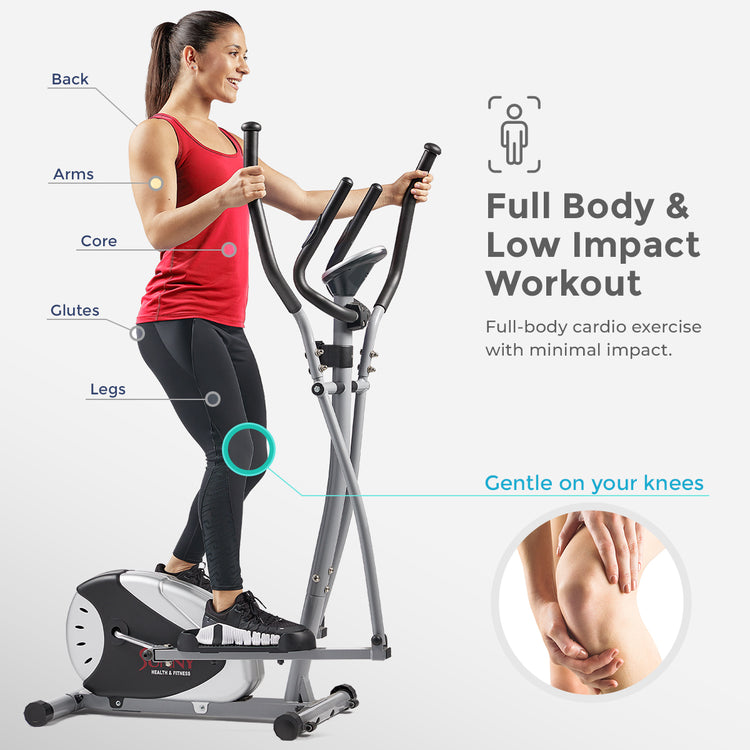The square image with a light gray background appears to be an advertisement promoting elliptical workouts, emphasizing a full-body and low-impact exercise. It measures approximately six inches by six inches. On the left-hand side, a woman with light tan skin and long brown hair tied back in a ponytail is using a small black and gray elliptical machine. She stands straight, facing right, with a smile on her face, wearing a red tank top, black leggings or yoga pants, and black shoes. Her left arm is extended, and her right arm is bent at the elbow. 

Various parts of her body – back, arms, core, glutes, and legs – are labeled with lines indicating the exercise benefits of the machine. A circle around her knees highlights that the elliptical is gentle on the knees. On the right-hand side, gray text reads, "Full body and low impact workout," followed by, "Full body cardio exercise with minimal impact." There is also a notable circle in the lower right-hand corner with a white background, showing a person grasping their knee, reinforcing the point that the machine is gentle on the knees. The depiction of the woman and the accompanying labels collectively convey the advertisement's message that the elliptical provides a comprehensive, yet gentle workout.